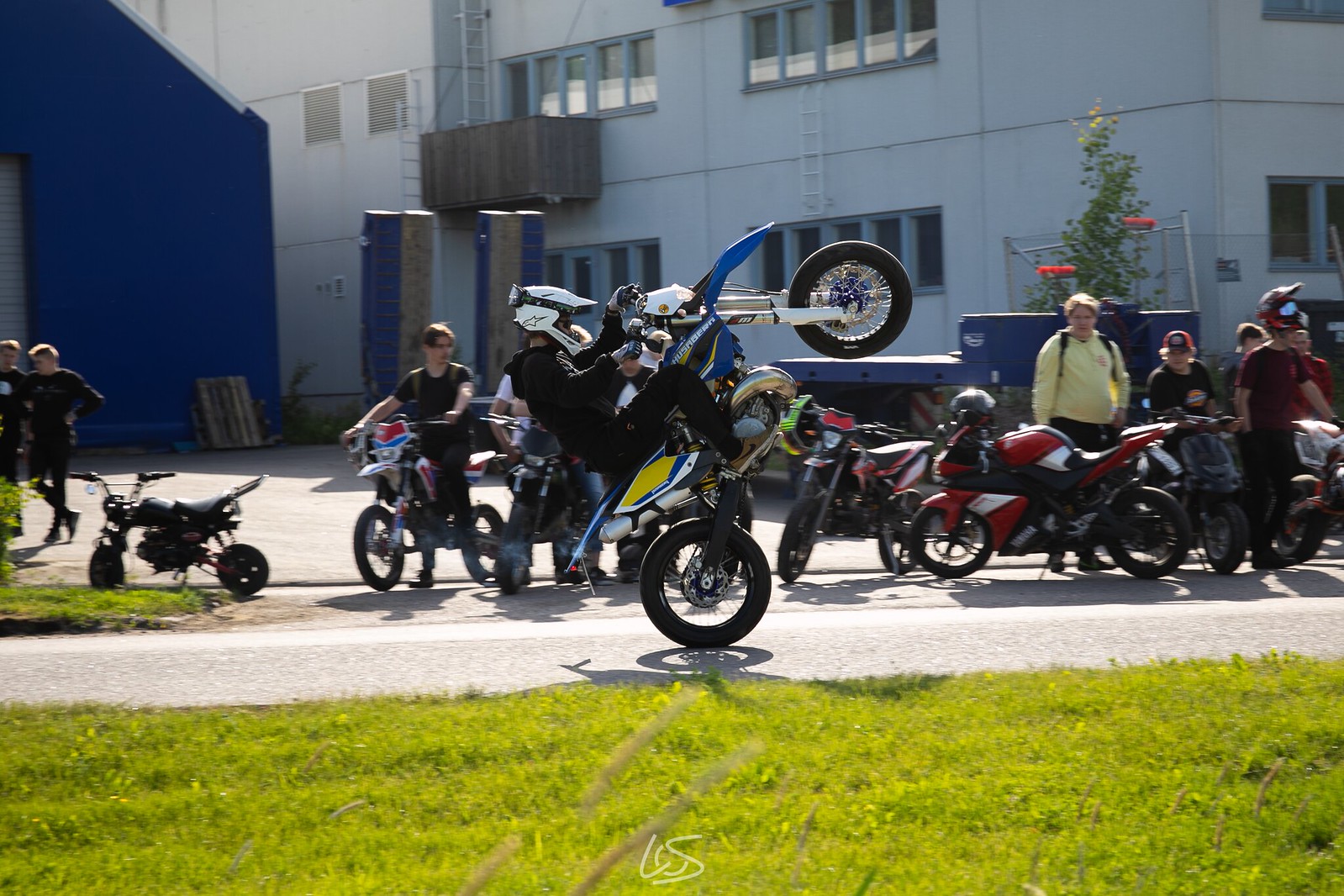The image depicts an outdoor scene in front of a large white warehouse building with a smaller, dark royal blue warehouse to its left. In the middle foreground, a man in a white helmet and all-black attire performs a wheelie on a blue and yellow dirt bike, its front tire lifted off the pavement. The grassy area at the front transitions into pavement where the action takes place. Around the man, approximately ten spectators stand or sit on various motorcycles, predominantly dirt bikes. Among them, a woman in a large yellow sweatshirt with a backpack stands out. Further left, a small minibike, suitable for a child, is visible. A blue flatbed trailer is parked in front of the white warehouse, adding to the busy, vibrant atmosphere of the scene.